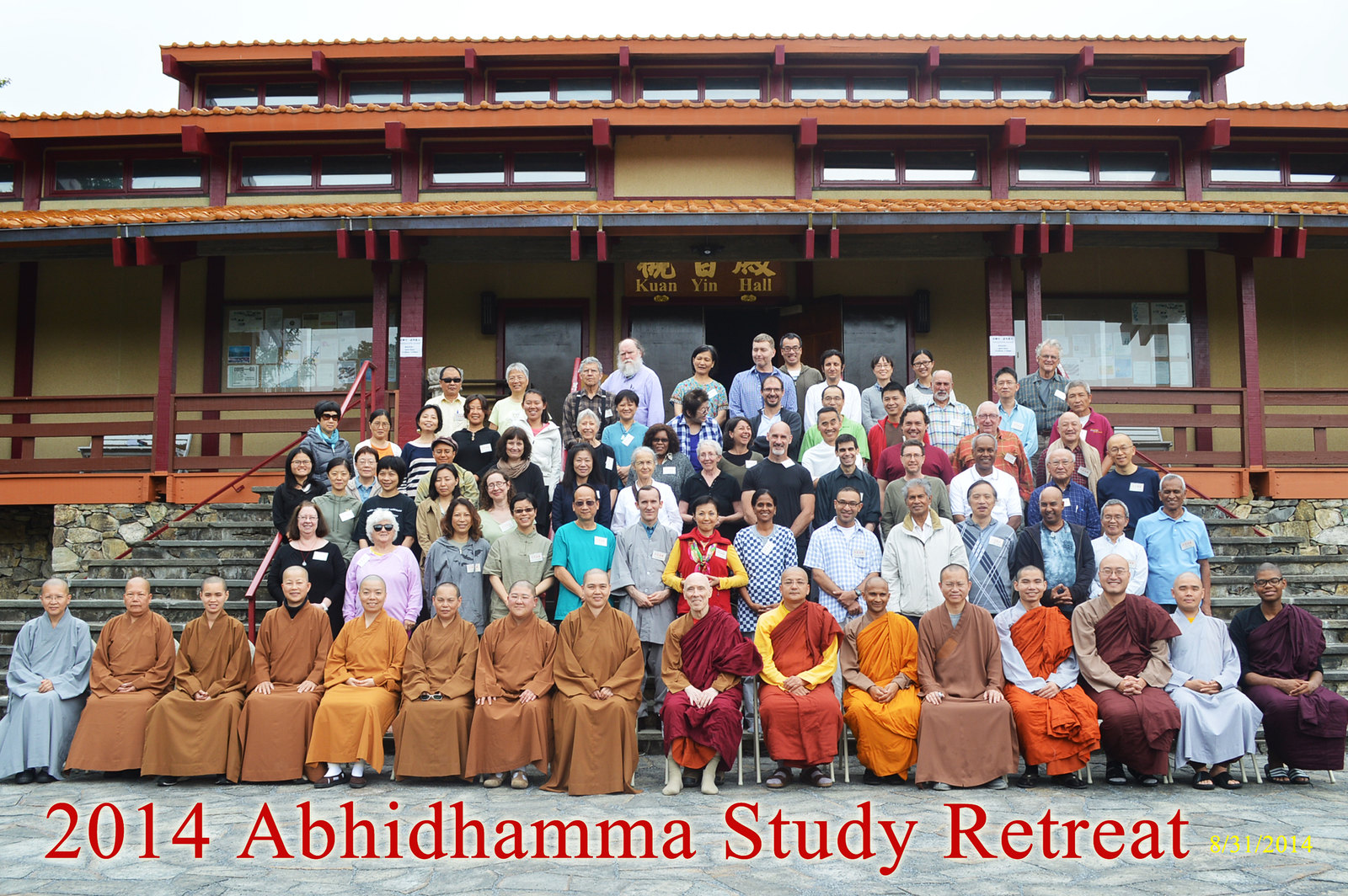In this vibrant color photograph, a large group of people is gathered on the cement steps outside a traditional Buddhist temple, identified as Guanyin Hall. The temple features beige walls and an orange terracotta roof, tiered into three levels, creating a striking backdrop. The image is captioned in red with "2014 Abhidhamma Study Retreat" and dated in yellow, "8-31-2014."

In the front row, several Buddhist monks are seated, distinguished by their shaved heads and an array of robes in brown, red, orange, and blue. These monks have their hands clasped or resting in their laps, exuding reverence and tranquility. Behind them, several rows of diverse participants stand on the steps, many adorned with name tags. The attendees display a colorful variety of attire, contributing to the lively and inclusive atmosphere of the event. The image captures a moment of unity and shared learning, set against the serene and spiritual backdrop of the temple.